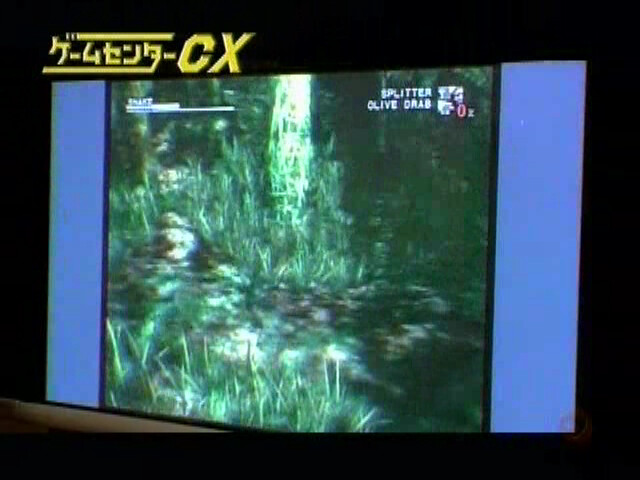The image appears to be a photograph of a screen, possibly from a TV or old camcorder. The screen has blue columns on each side and a black border surrounding the central image. The photograph itself features an outdoor forest scene, focused on the ground, with a tree and some tall grass visible. The quality is blurry, reminiscent of VCR footage from the 1980s.

In the top left corner of the image, there is small, unreadable text. In the top right corner, the word "SPLITTER" is displayed in all caps, and below it, also in all caps, is the phrase "OLIVE DRAB." Accompanying these words is an image of a woman, displayed in red, along with a red symbol that appears to be a zero or a letter "Z," colored gray. At the very top of the screen, yellow text is shown in an Asian script, and to the right of this text is the phrase "-CX" in large letters.